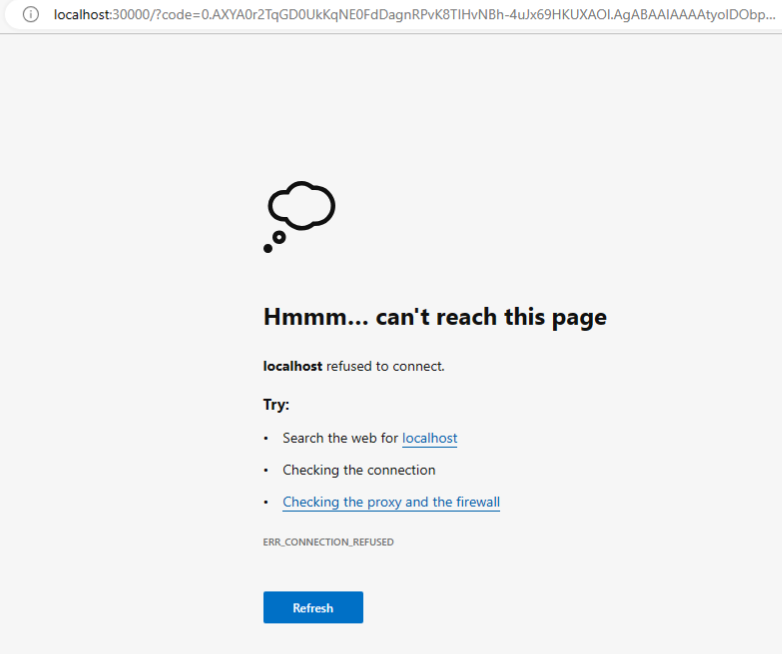The image features several elements arranged in a specific layout. At the top, there is an oval-shaped white search box, which appears truncated on the right side. This search box has a gray outline of a circle on its left side, containing a white background with a gray lowercase "i" inside. The text within the search box is black, reading "localhost," followed by grayed-out characters: "...,300/?code=0.AXYA0R2TQGD0UKKQNE0FDDAGNRPVKATI-VN-BH-4UJXCXVOVKATI-VN-BH-4UJXCXVOVKATI-VN-BH-4UJXCXVO..." and so on.

Below the search box, the background shifts to gray, showcasing a prominent black cloud icon. Underneath this icon, in bold black text, the message "Hmmm... Can't reach this page" is displayed. Further down, additional text states: "localhost refused to connect." This is followed by suggestions in black text: "Try... Searching the web for localhost... Checking the connection... Checking the proxy and firewall settings."